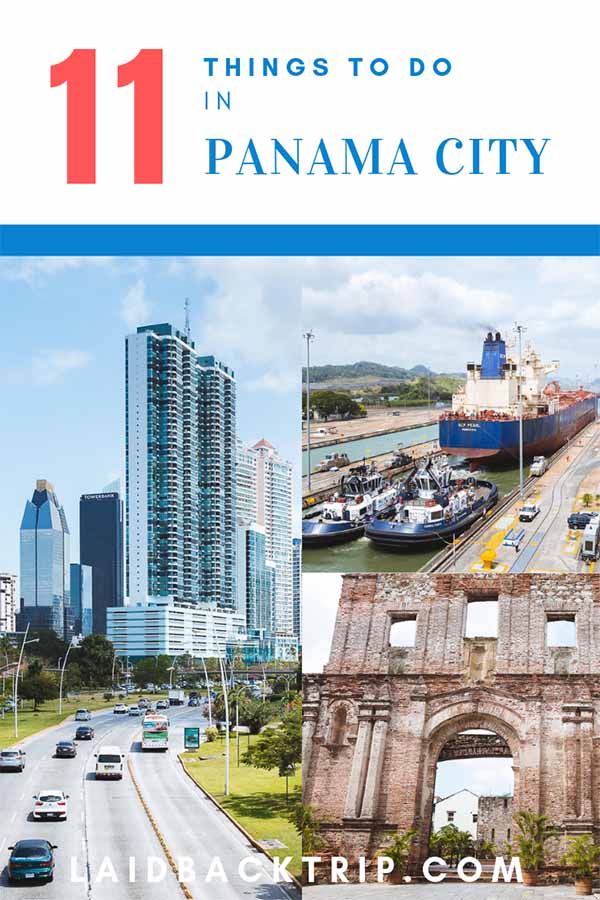The image prominently features an advertisement or promotional photograph titled "11 Things to Do in Panama City," with "11" showcased in a large, striking red font, while "Things to Do in Panama City" appears in a vivid blue font to its right. The layout includes three distinct photographs that capture diverse scenes of the city.

On the right side of the image, a large photograph offers an aerial perspective of a bustling highway, suggesting a drive through Panama City’s urban landscape. In the top right corner, a smaller image displays three sizable boats docked between two roads, hinting at the city's vibrant waterfront and maritime activity. The bottom right photograph presents an intriguing view of what appears to be a medieval-style ruin or historic building, evoking a sense of the city’s rich historical tapestry.

At the bottom of the image, the website "laidbacktrip.com" is inscribed in clean white font, guiding viewers to visit the site for more information. The composition of the image provides a multifaceted glimpse into the attractions and experiences awaiting visitors in Panama City.